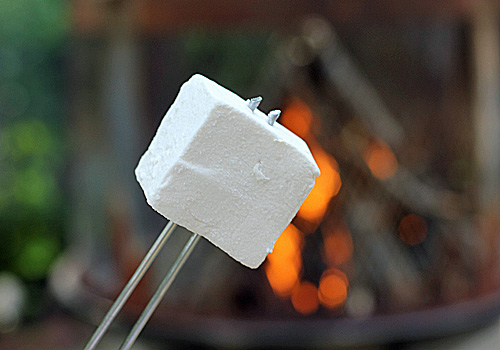The image depicts a pair of metal tongs, comprised of two pointed metal wires, emerging from the bottom left and angled diagonally to the top right. The tongs are sharply in focus, holding a white, square-shaped object that has a marshmallow-like texture, though it could also be cheese or tofu. Visible at the ends of the tongs, the metal tips slightly protrude from the top of this mysterious food item. In the blurry background, there appears to be an outdoor scene with a campfire made from stacked wood, glowing with orange and yellow flames. The surrounding green foliage suggests that the setting is likely a campground, with hints of trees or bushes blending into the backdrop. The fire seems to be contained within a circular fire pit, as indicated by a visible rim at the bottom of the stacked wood. The overall scene suggests that the object on the tongs is intended for cooking over the campfire.